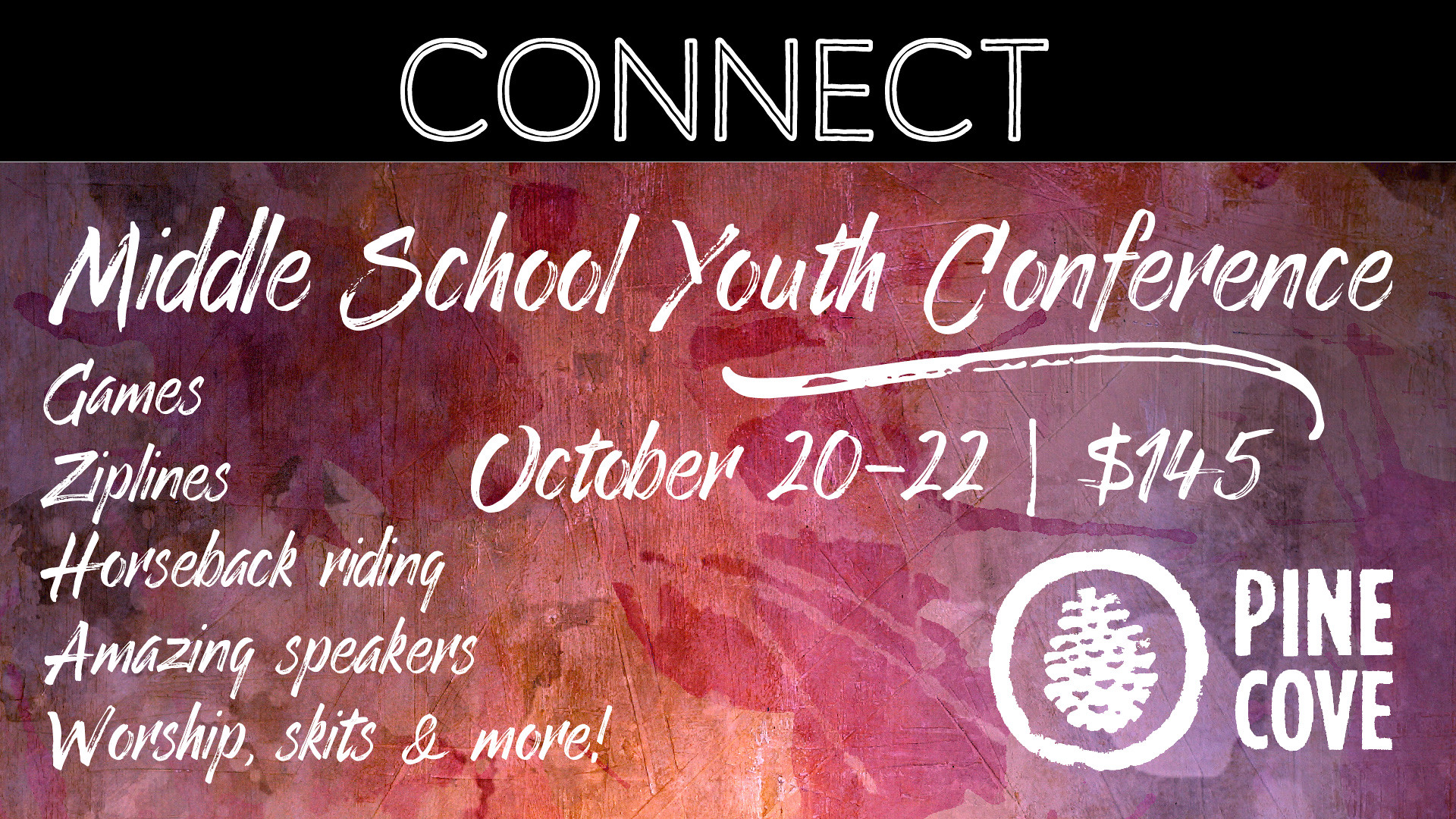This image is a horizontal advertisement for an event, primarily dominated by a color scheme of purples, reds, and oranges, reminiscent of a watercolor splatter. At the top is a striking black bar that spans the width of the image, where the word "CONNECT" is prominently displayed in large white capital letters. Below this bar, against the artistic, leafy background, the details of the event are announced in white chalk-like cursive font. It reads "Middle School Youth Conference," followed by an enticing list of activities including games, zip lines, horseback riding, amazing speakers, worship, and skits. The event spans from October 20th to October 22nd, 2020, with a participation fee of $145. In the bottom right corner, the logo of Pine Cove is featured, consisting of a white pinecone encircled within a white border, accompanied by the words "Pine Cove" in block letters. This comprehensive flyer thus serves as an informational sheet detailing the essential aspects of the upcoming middle school youth conference.